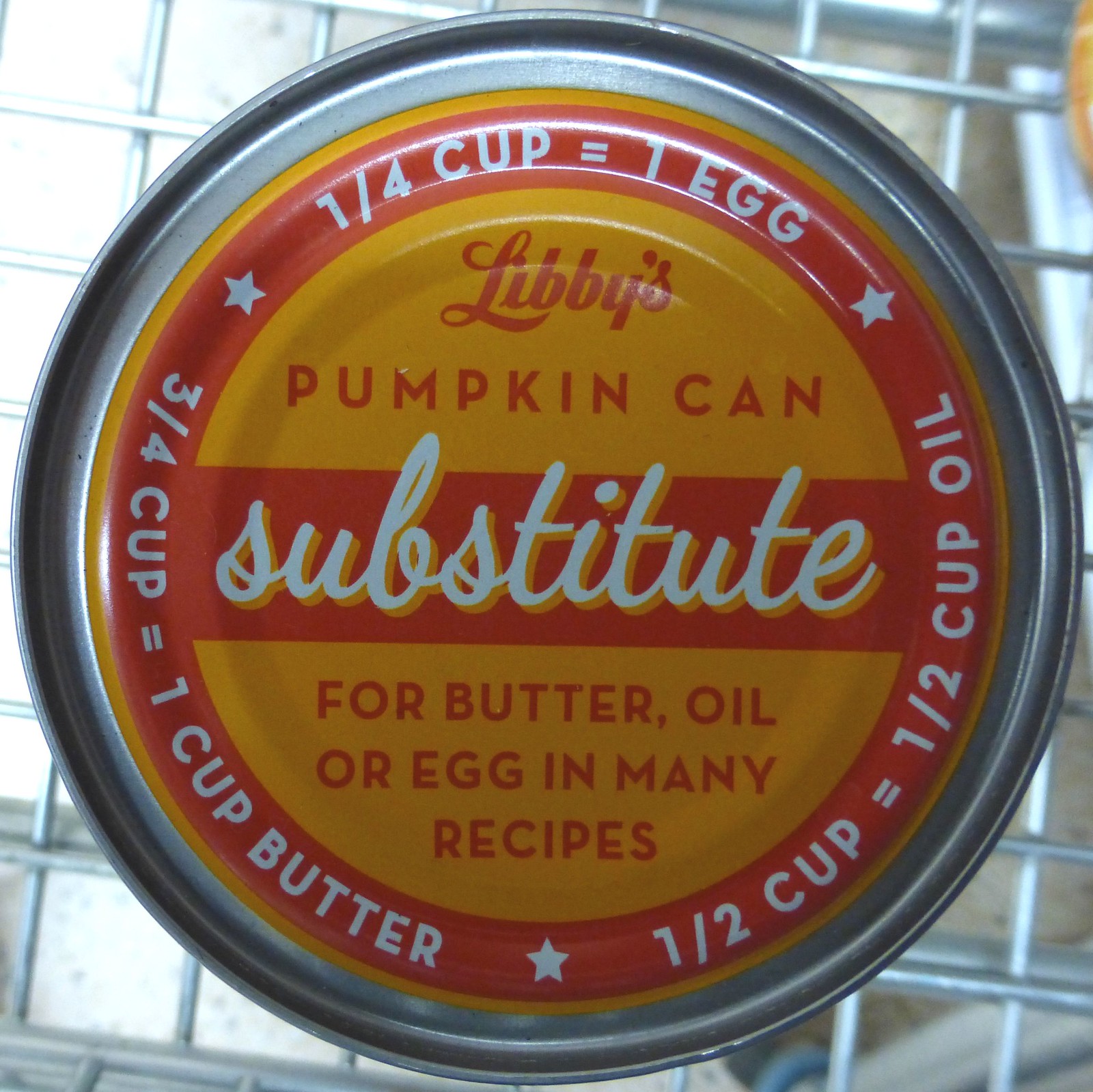This image features the lid of a Libby's Pumpkin Can, resting on a metal grate shelf. The lid has a circular logo design with an orange background and a prominent red border. At the top of the circle, the text reads "Libby's Pumpkin Can" in a bold, red font. Below that, a red stripe runs horizontally through the middle of the circle with the word “Substitute” elegantly scripted in white cursive. The text at the bottom of the circle reads, "for butter, oil, or egg in many recipes" in a clear, standard font. Encircling the text are substitution ratios surrounded by small stars for visual emphasis: "1/4 cup equals 1 egg," "1/2 cup equals 1/2 cup of oil," and "3/4 cup equals 1 cup of butter." The cohesive design in shades of orange, red, and yellow is eye-catching and informative, providing useful culinary tips right on the can lid.